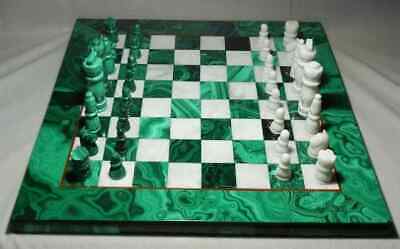The image features an exquisitely designed chessboard resting atop a pristine white sheet or blanket. The border of the chessboard is crafted from a luxurious, green marble-like gem, giving it a refined and elegant appearance. The checkerboard pattern consists of alternating squares of white and an iridescent jade green, enhancing the board's visual appeal. The chess pieces are positioned in their starting placements: the set on the far right are pure white, while the pieces on the left mirror the board's border with their matching jade green color. No moves have been made, and the scene is characterized by an untouched, ready-for-play feel. In the corner of the image, there's a small dot with a camera icon, subtly indicating the photograph's origin.